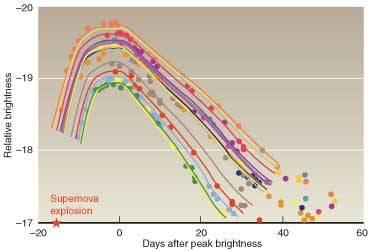This detailed square image showcases a colorful line graph with a dark pinkish beige background. The y-axis, labeled "Relative Brightness" in black letters, ranges from 17 to 20. The x-axis, titled "Days After Peak Brightness," spans from negative 20 to 60. At the bottom right corner of the graph, there is a red-printed label, "Supernova Explosion," marked with a star at the point negative 20. The graph features multiple colored lines—red, yellow, purple, black, green, and blue—each depicting data points that form a wave-like pattern. These lines rise sharply and then decline more gradually as they extend toward the right, forming a dynamic visual representation with dots marking specific data points along the way.